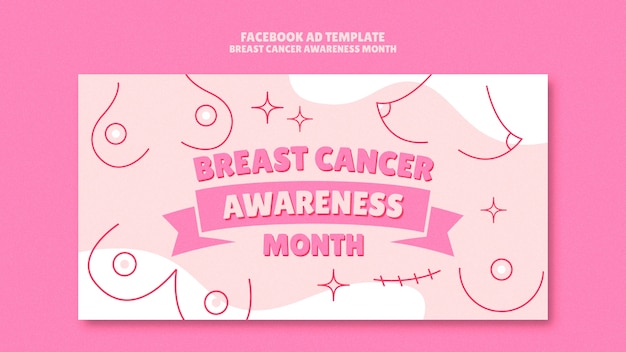The image is a poster designed as a Facebook advertisement template for Breast Cancer Awareness Month, framed with a pink border at the top. The central graphic prominently states "Breast Cancer Awareness Month" with the words "Breast Cancer" and "Month" displayed in pink, while "Awareness" is inscribed within a pink ribbon. The poster features a series of computer-generated illustrations of breasts, depicted in simple lines and various shapes to represent diversity. Additionally, there are decorative four-pointed stars scattered throughout the design. Notably, the image includes a stitching-like element, symbolizing surgical incisions related to breast cancer treatment, rendered in a beige color to invoke a medical context.